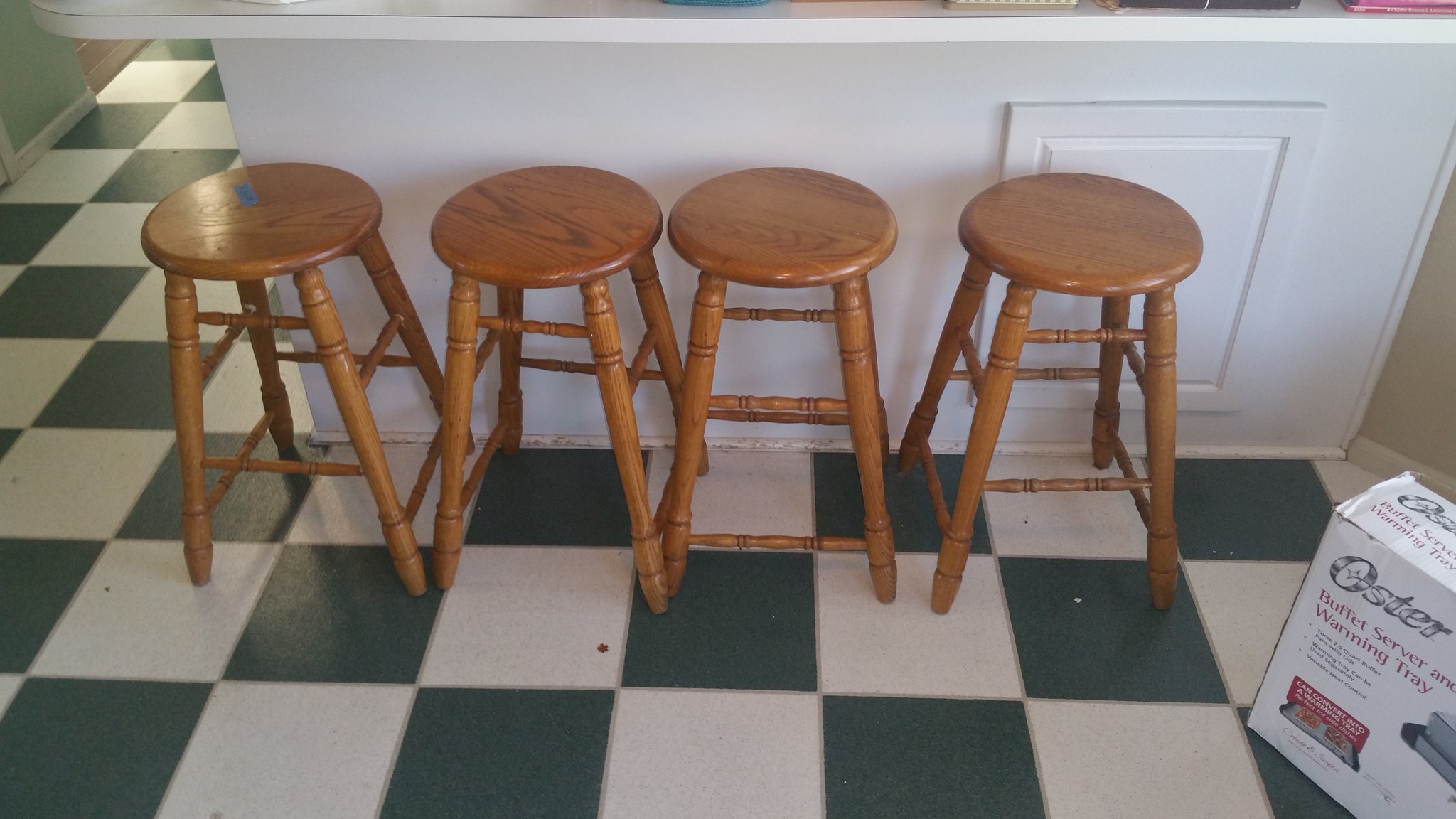In this image, we see an indoor kitchen setting dominated by a large white bar with a Formica top and a curved corner. Arranged neatly in a row directly across from the bar are four medium wood stools, their finished surfaces gleaming in the light. The leftmost stool has a piece of blue gaffer's or painter's tape attached to it. The floor beneath is a striking dark green and white checkerboard pattern, continuing under the bar’s left corner where a light green wall with white trim and the entrance to a doorway can be seen. To the right of the stools, a white box for an Oster buffet server and warming tray sits on the floor, partially opened and revealing that it is a 2.5-quart appliance. Directly above the rightmost stool, a small panel likely provides access for plumbing, hinting at a sink just out of view. The setting suggests a cozy, functional kitchen area perfect for gathering.